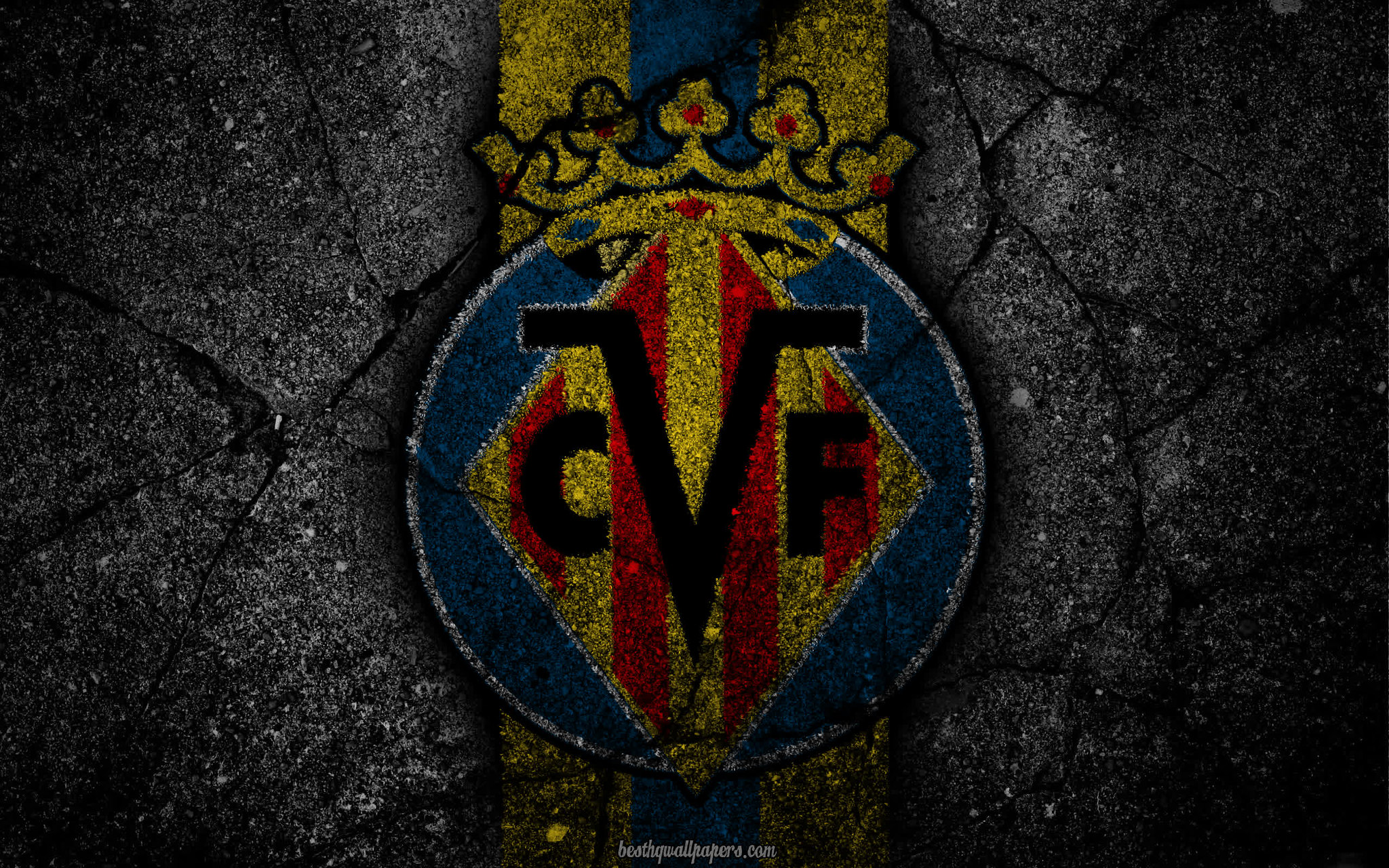The image showcases an emblem painted onto a cracked, dark-gray asphalt surface with black flecks. At the core of the emblem is a blue circle with a white outline, containing a prominent yellow and red horizontally-striped diamond. Within the diamond, the letters "CVF" are inscribed in black, with the "V" noticeably larger than the "C" and the "F" on either side. At the top of the circle, a yellow crown is perched, adding a regal touch. Flanking the circle at the top and bottom are vertical stripes of yellow, blue, and yellow, resembling watch bands. The entire design appears embedded into the weathered pavement, giving it a rugged, urban character.